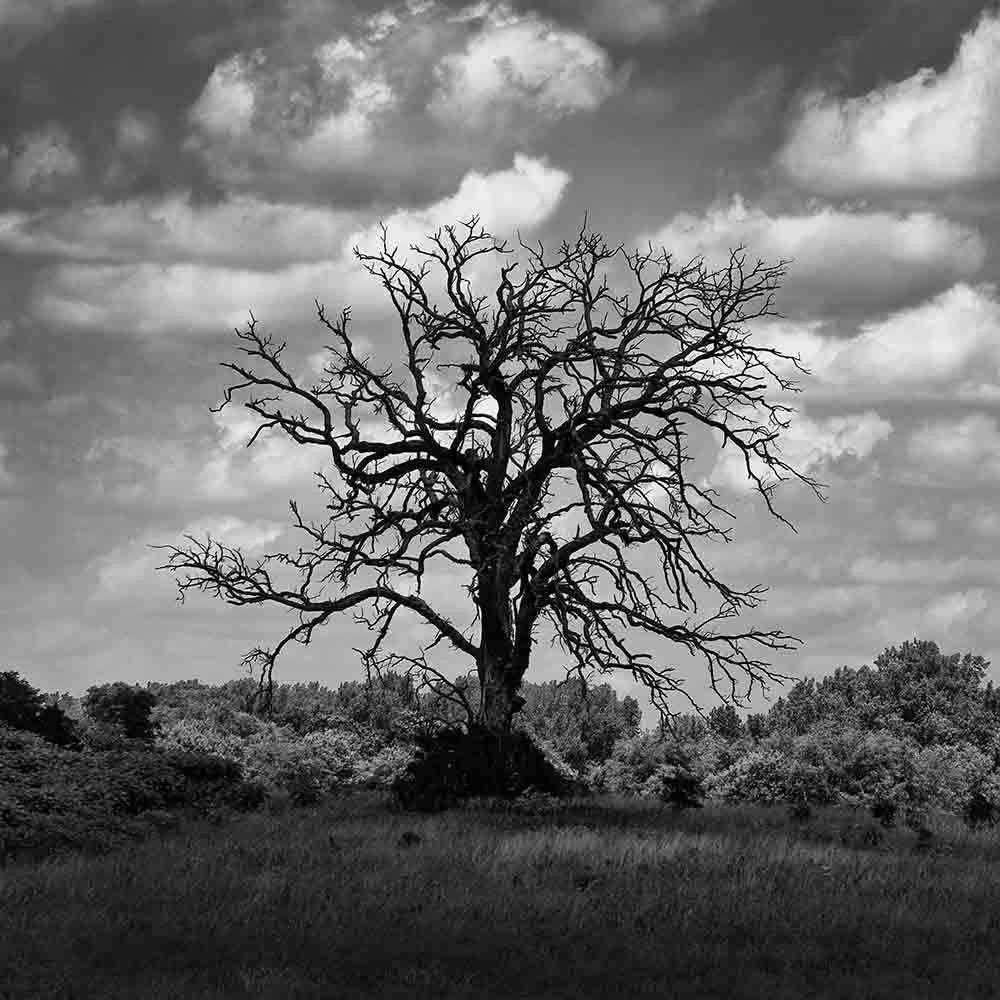This black and white photograph, approximately 6 inches square, captures a starkly barren tree centered in a grassy field during the daytime. The sky above is a cloudy mix of grays and whites, casting a somber mood over the scene. The tree, standing about 40 to 50 feet tall, has an intricate network of branches sprawling in all directions, devoid of any leaves. Surrounding the tree at its base are patches of dark shrubs, adding to the textured shadow that creeps from its roots. Beyond this central tree, more vegetation is visible, with a mix of smaller shrubs and taller tree tops creating a layered backdrop of varying gray tones. The entirety of the setting is enveloped in the grayscale palette, stripping away any hint of color, thereby emphasizing the bleak beauty of the landscape.